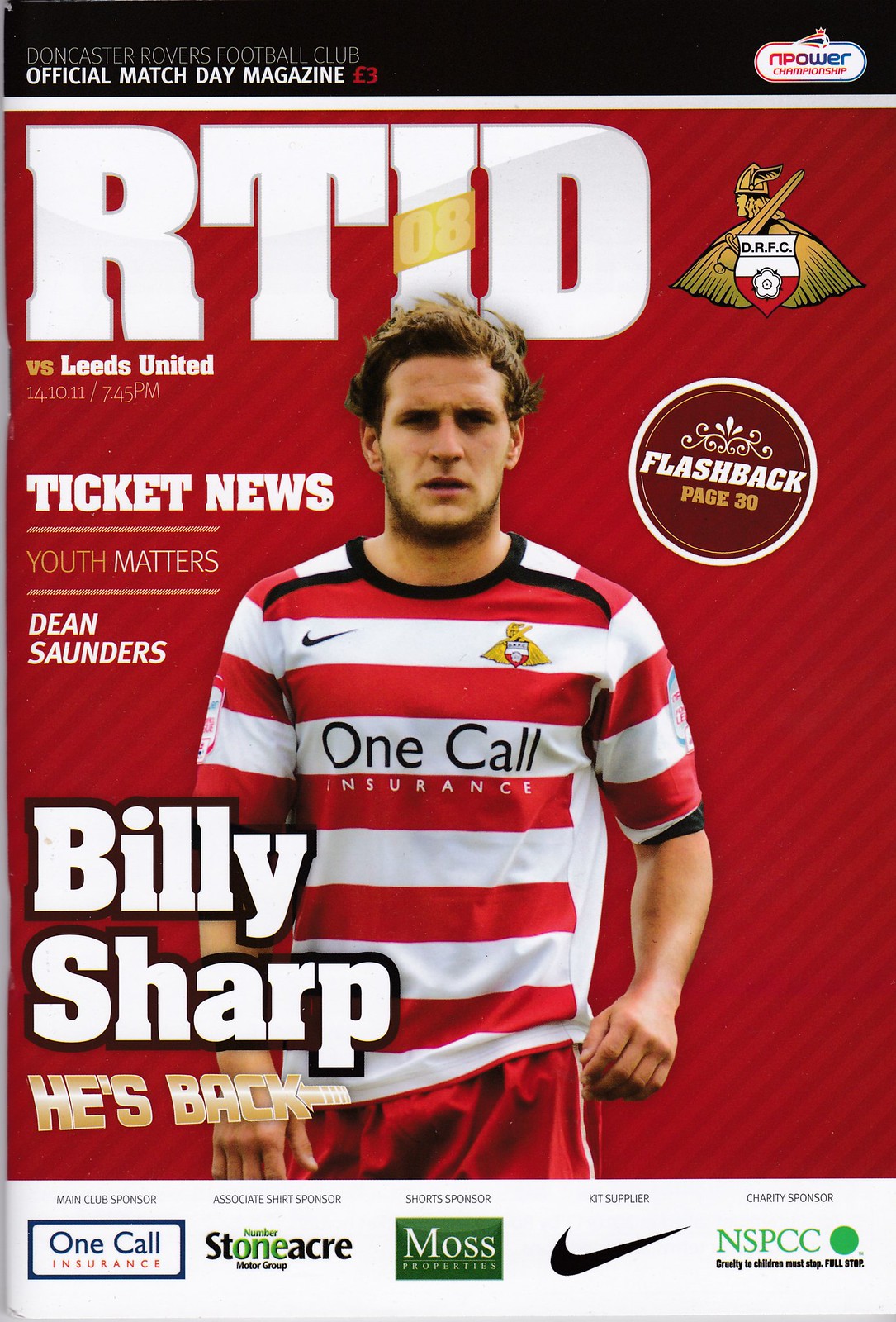This vertically aligned, rectangular image depicts the cover of an official match day magazine from Doncaster Rovers Football Club, priced at €3. The top section features a black border with the text "Official Match Day Magazine" and beneath it, a logo with "Npower Championship". A white horizontal line separates this from the main cover, which has a red background with subtle diagonal stripes. Dominating the cover is the large, white block letters "RTID" in the upper left corner, with a gold "08" across the 'I'. 

A prominent football player is centered on the cover, wearing a red and white striped jersey emblazoned with "One Call Insurance" and the Nike logo, paired with red shorts. He has brown hair, some facial hair on his chin and cheeks, and an assertive stance. To the left of the player, headline sections read "Ticket News", "Youth Matters", and "Dean Saunders", all in white capital letters. 

On the upper right, the DRFC logo featuring a gold image of a figure with a sword is visible, accompanied by a circular area with the text "Flashback Page 30". At the lower left corner, bold white text outlined in black proclaims "Billy Sharp", followed by "He's back". The bottom section of the cover displays logos of sponsors, including Nike, Moss, and NSPCC.